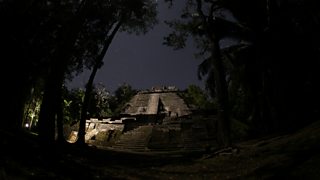The small, dark, rectangular image appears to be taken at nighttime, making it challenging to discern specific details. The scene features numerous trees on both the left and right sides, surrounding what seems to be an old stone or concrete structure. This structure might be a building or monument, characterized by steps leading up to a platform. A light source, possibly from a car, streetlight, or spotlights, illuminates part of the structure from the left. The sky above is a solid gray, adding to the dim, shadowy ambiance of the photo. Despite the low visibility, the composition hints at an eerie, forested area with a historic or ancient feel.